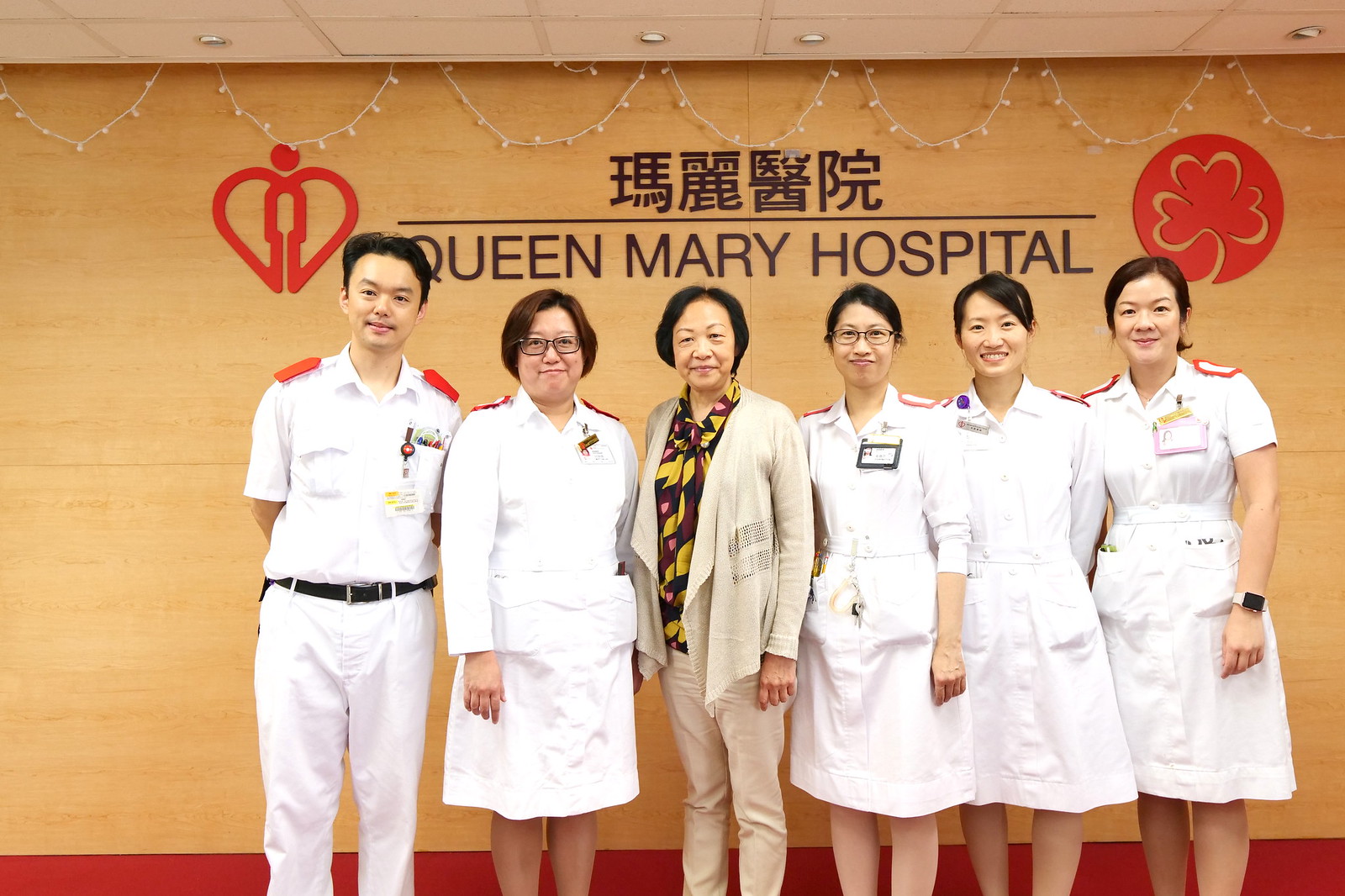This photograph features a group of six Asian individuals standing in front of a wall with the text "Queen Mary Hospital" in both English and Chinese characters. The backdrop is light brown and includes two distinct logos: a heart with a person in the center on the left, and a three-leaf clover-like design on the right. The group comprises one man and five women, all dressed in medical attire, except for one woman in business attire. 

The man, positioned on the far left, wears a white uniform with orange shoulder pads and a name tag, and has pens in his front pocket. The three women on the right wear matching white medical dresses with name tags and shoulder patches, with the second woman from the right also sporting glasses. The woman at the center is dressed in a beige over shirt and beige pants, making her stand out as she is in business attire. All individuals are facing and looking at the camera, giving a professional and cohesive appearance.